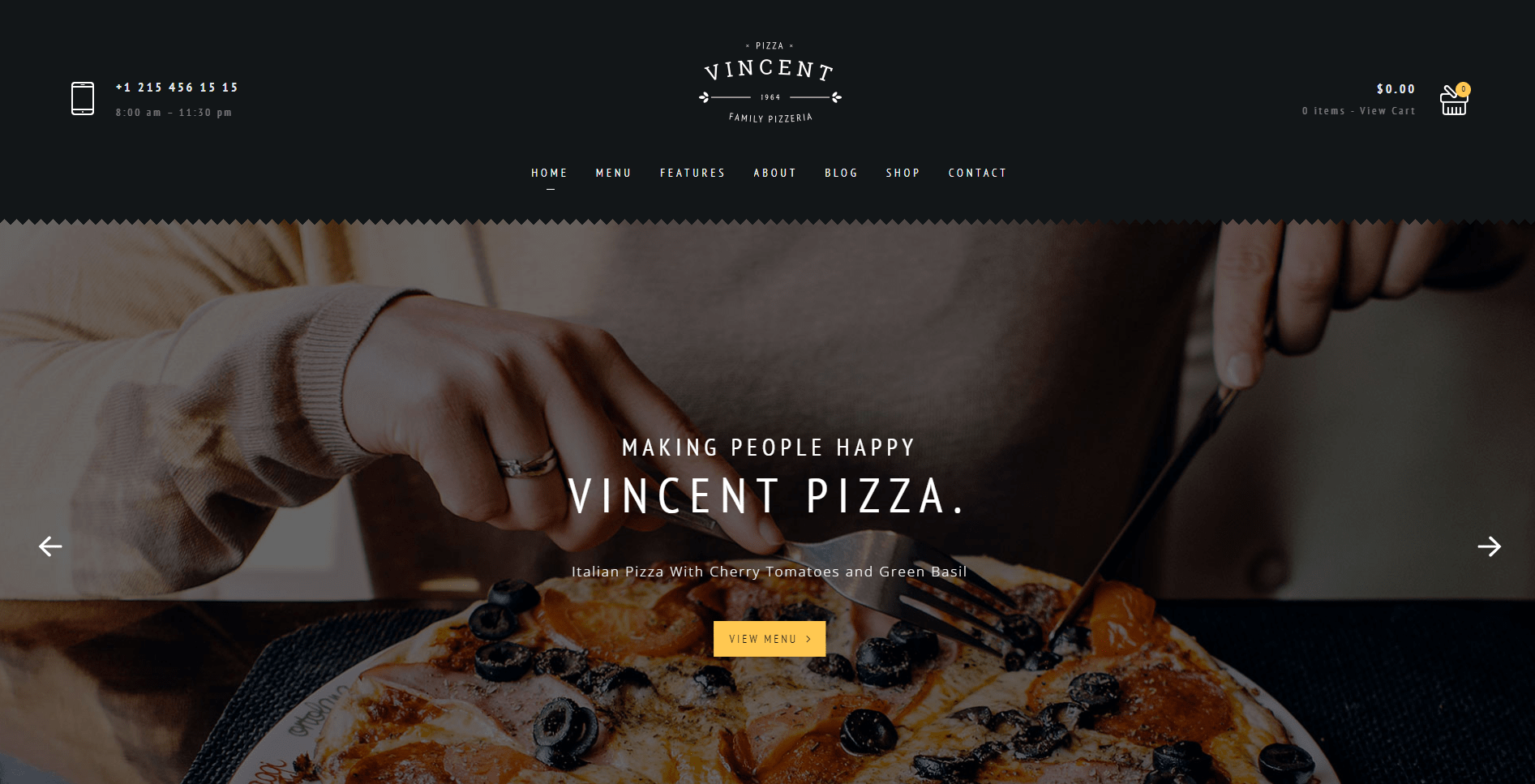This horizontal image showcases the homepage of a restaurant's website, accessible via computer or smart device. The restaurant, likely a pizza or Italian eatery, features a clean, flat black background at the top of the page. 

On the left side, there's a small white phone icon displaying the contact number and operating hours in gray (8 a.m. to 11:30 p.m.). Centrally positioned is the text "Pizza Vincent Family Pizzeria 1964" in white. Below this, the navigation menu includes options for Home (underlined to show it is selected), Menu, Features, About, Blog, Shop, and Contact. 

On the upper right-hand side, the site shows an empty shopping cart indicated by "0.00, Zero Items, View Cart" along with a cart icon that has a zero inside an orange circle. 

The main background picture features a person cutting into a pizza. Only their hands and part of their shirt are visible, focusing the viewer’s attention on the knife, fork, and the pizza itself. Overlay text reads "Making People Happy, Vincent Pizza, Italian Pizza with Cherry Tomatoes and Green Basil," accompanied by a prompt to "View Menu."